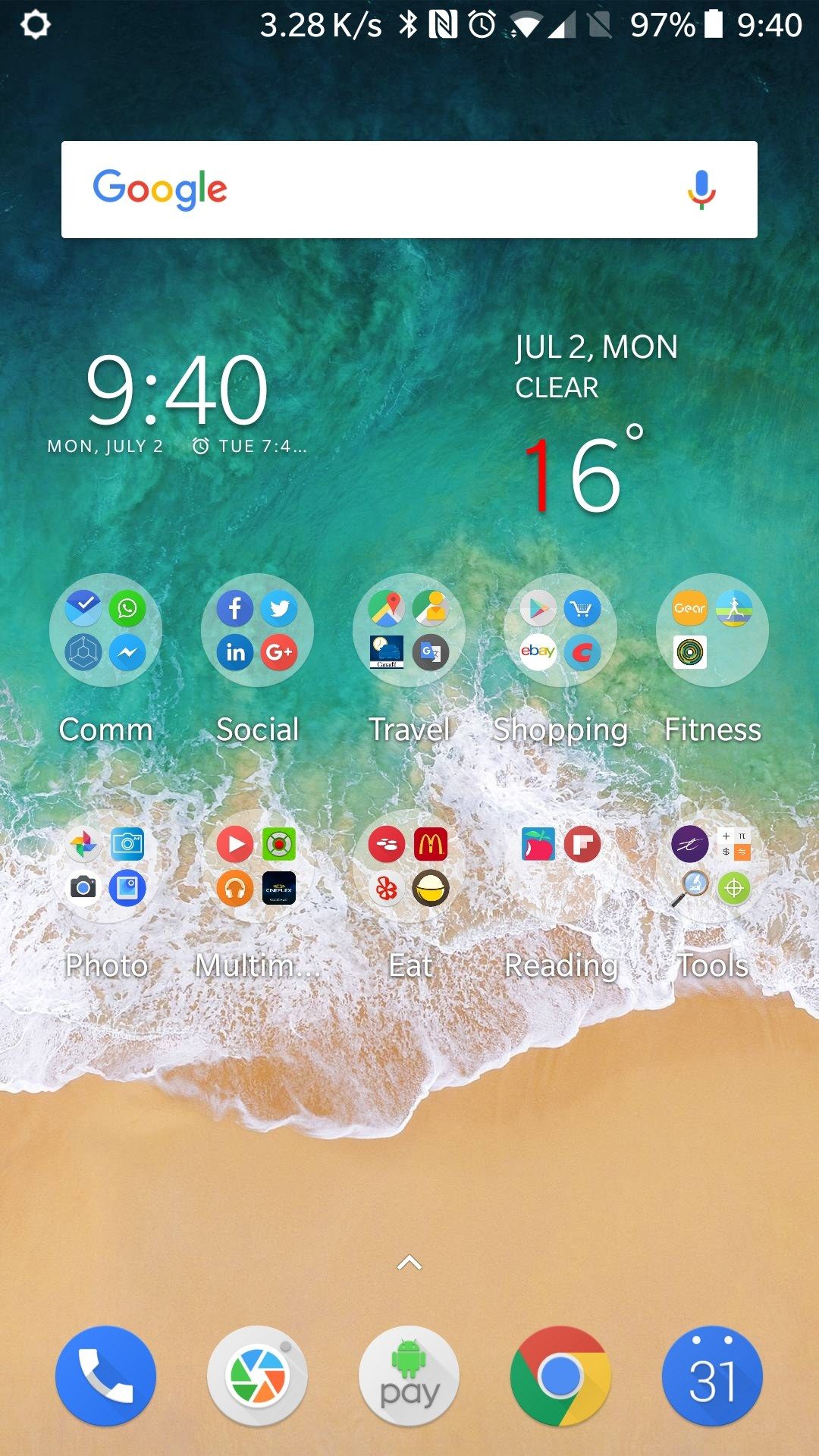This image is a detailed screenshot of a smartphone home screen, showcasing various elements in a well-organized manner.

At the very top, the status bar, rendered in a dark greenish-gray shade, displays crucial information. On the right side, in white font, the time reads "9:40." Next to it, a battery icon indicates a 97% charge. A series of icons follow, representing the wireless signal, Wi-Fi, alarm, and Bluetooth. Additionally, a speed indicator reads "3.28 K/s."

Beneath the status bar, the prominent Google search box sits as a white rectangle. On the right side of the search box is a microphone icon, suggesting voice search capability. To its left, the familiar Google logo appears, with a blue 'G', red 'O', yellow 'O', blue lowercase 'g', green 'l', and red 'e.'

The background image is a serene beach scene. At the bottom, the sandy beach transitions to the tide, with white surf moving into varying shades of green water that darken towards the top.

Below the search box, the time is displayed again, "9:40," in white font. Accompanying this on the right side, the date reads "July 2, Mon," with weather information indicating clear skies and a temperature of 16 degrees.

Further down are two rows of app folders. Each folder is represented as a circle with a light blue background and contains various app icons. Notable apps include Facebook, LinkedIn, Google+ (indicating the screenshot's age), and YouTube among others.

At the very bottom of the screen, four essential app icons are easily accessible: Phone, Android Pay, Google Chrome, and Calendar.